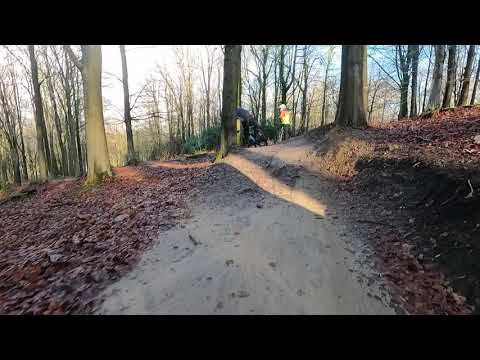This photograph captures a serene landscape featuring a forest trail flanked by tall, medium-thickness trees with green moss. The dirt path, speckled with fallen reddish-brown leaves and occasional sticks, runs straight before curving slightly to the right around a sloping hill. The scene includes two large trees prominently positioned alongside the trail and several smaller ones dispersed throughout. In the distance, a person wearing a yellow and orange top with a white helmet or light-colored hair stands facing left, adding a focal point of interest. The sky above is a mix of blue patches and white clouds, hinting at a mildly cloudy day. Shadows from the trees stretch across the pathway, enhancing the depth and tranquility of the woodland setting. The image is framed by black bars at the top and bottom, giving it a cinematic quality.